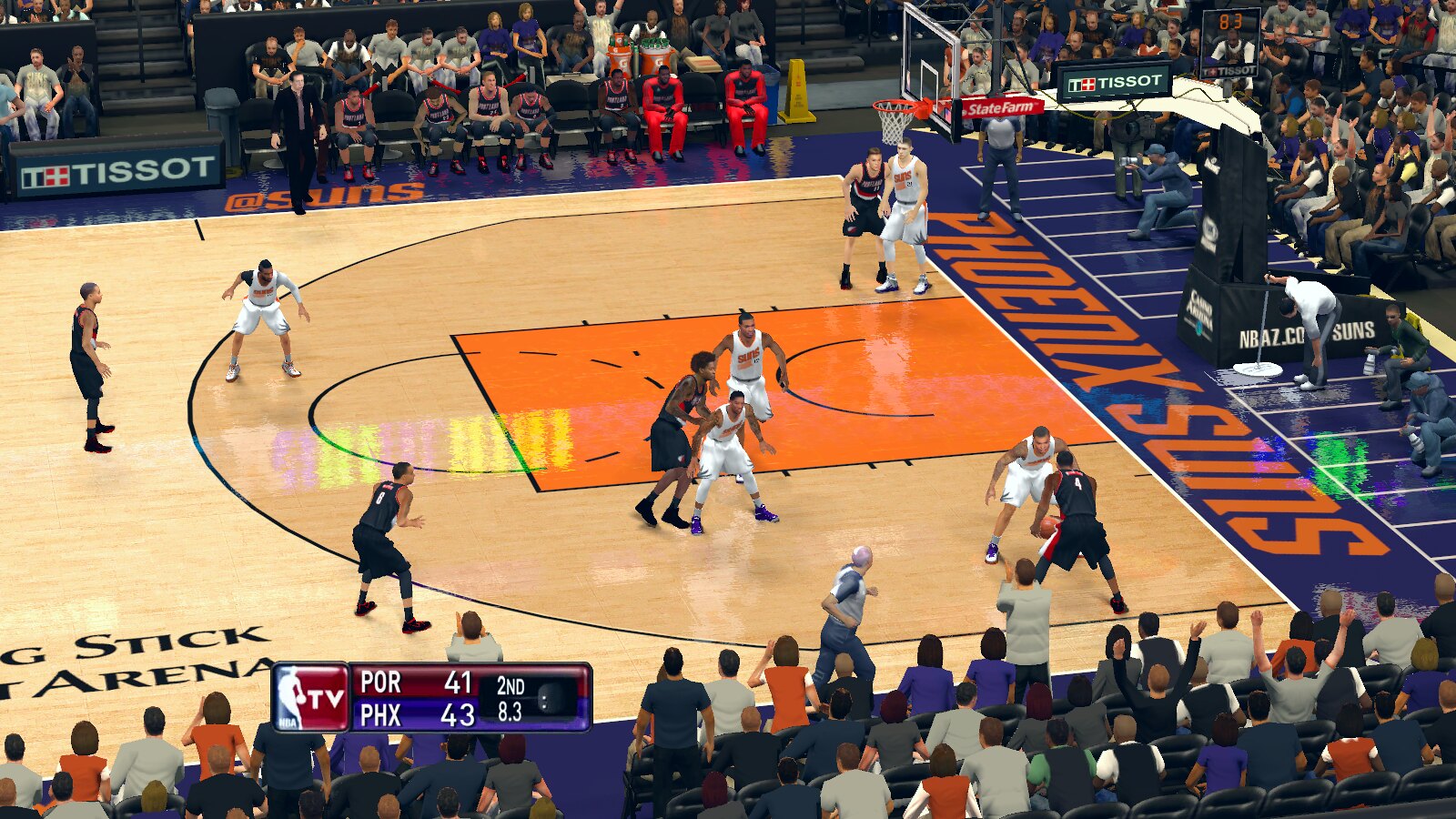Captured from a vantage point in the bleachers, this image provides a bird's-eye view of an intense basketball game unfolding on the court below. The focus is drawn to a digital scoreboard in the lower left-hand corner displaying the current score: POR leads with 41 points while PHX is closely trailing with 43 points. The game is in its second period, with only 8.3 seconds left on the clock for this half. On the court, players are strategically positioned, and one player in the lower right is notable for having possession of the ball, presumably preparing to make a crucial play. The seating area is filled with spectators, creating a dynamic and exciting atmosphere as the game progresses.